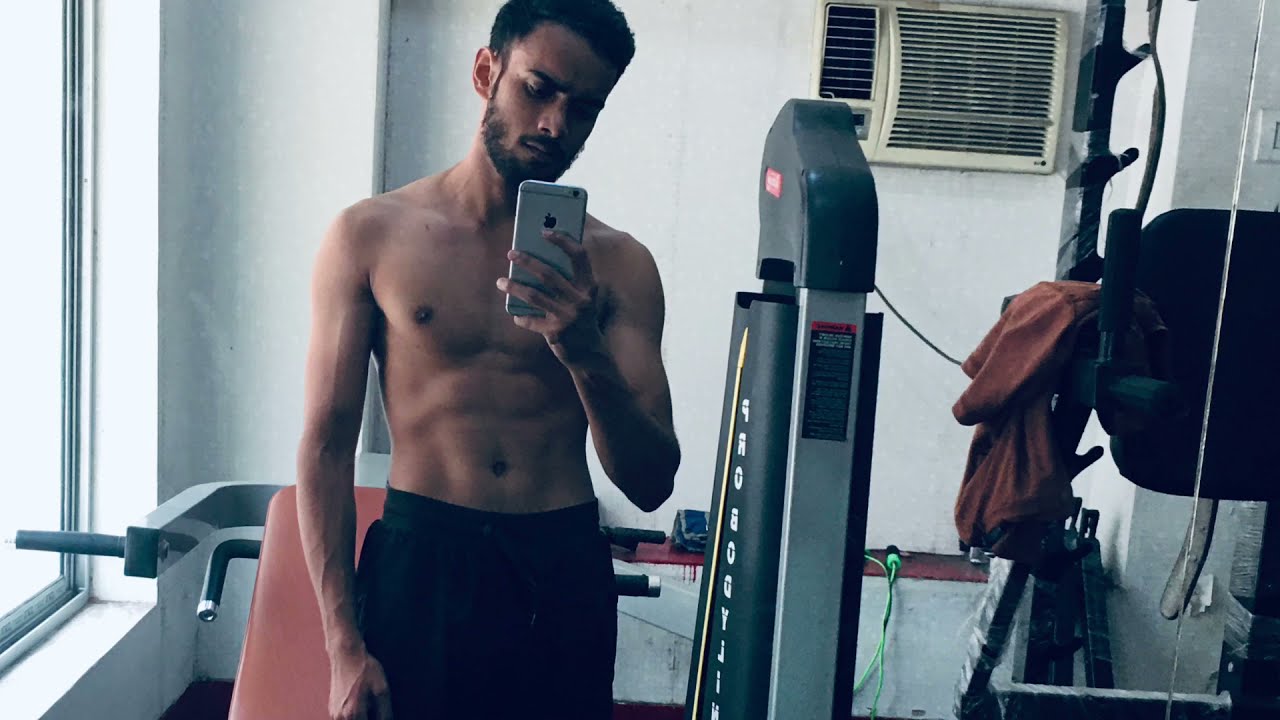In an indoor gym with white walls, an air conditioning unit, and a large window on the left side, a man with light brown skin, short black hair, a black mustache, and beard is taking a selfie. He is shirtless, revealing well-defined muscles, particularly in his arms and abdominal area. The man, holding a mostly silver iPhone with his left hand, appears to be standing near a shoulder or chest press machine, which has a red backing and black handles. He's wearing black pants or shorts. Behind him on the left, there's a red bench with a green jump rope on it, and on the right, his red shirt is hung up on a piece of exercise equipment, likely a squat rack. The room is filled with natural light from the window, enhancing the overall scene of his workout space.